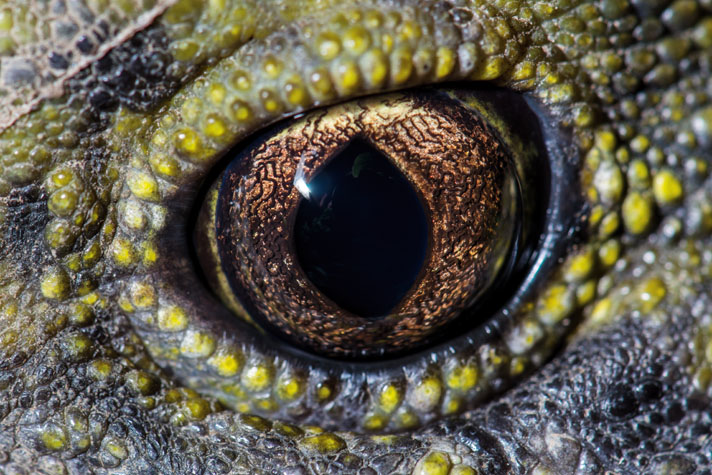The image is a highly detailed, close-up photograph of a reptile's eye, possibly belonging to a snake or lizard. The eye, taking center stage in the photo, is a deep bronze color with a large black pupil. Its iris is shaped somewhat like a teardrop, and the eye itself is wide open, lacking an eyelid. Surrounding the eye, the reptile's skin displays a mix of gray, yellow, cream, and green hues. The texture of the skin is dry and bumpy, covered in intricate beading and scaling patterns. The skin's many lines and indentations add to the very tactile, almost hyper-realistic appearance of the photograph. The overall scene conveys a distinctly unsettling, foreboding atmosphere, making the viewer feel as though the eye is staring directly at them with an eerie intensity.